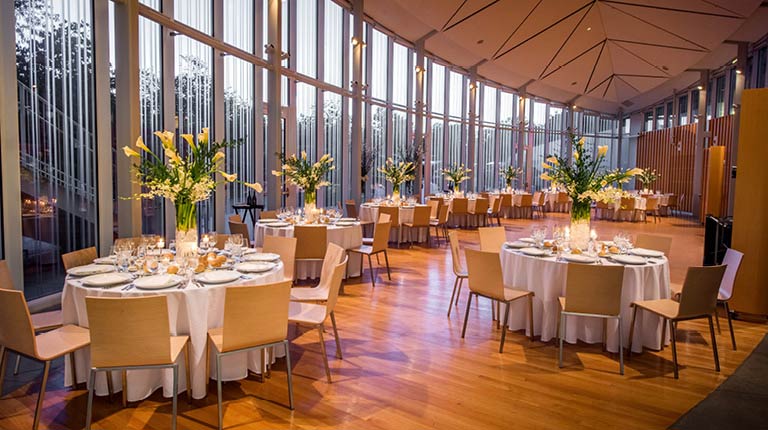This indoor color photograph, taken during the day, depicts a beautifully set up banquet or dining area with an elegant, circular-shaped room. The background features a curved glass wall with golden metal mullions, allowing light to stream through, although the exact outdoor view remains unclear. The tan hardwood flooring complements the light tan or muted pink tablecloths adorning multiple round tables that are closely arranged near the curved glass windows. Each table boasts a large, striking centerpiece of tall, likely yellow tulips or possibly white lilies with green stems in tall vases. The tables are set with white plates that have black trim, carefully arranged in a fancy dinner placement. The chairs surrounding these tables are a light, warm yellow or tan color, harmonizing with the overall decor. One distinctive ellipsoid table, presumably a head table, stands apart with its six chairs and non-circular shape. The room’s ambiance is further enhanced by a high brown ceiling with accent lighting, contributing to a sophisticated and inviting atmosphere.